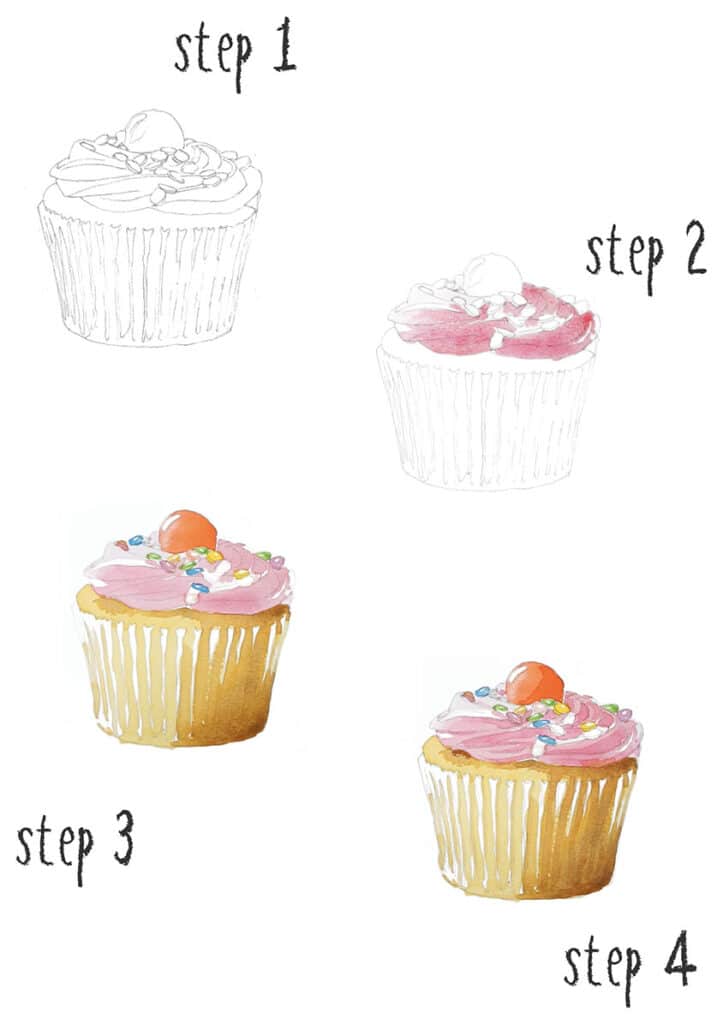The illustration is a detailed, step-by-step guide on how to color a cupcake. The image is divided into four steps, each labeled as "step" followed by a number, with the progression depicted through a series of drawings. 

In the first step, located in the upper left corner, the cupcake is shown in black and white, outlined in pencil. The cupcake features a ball-shaped fruit on top with small pieces of fruit and cream over a classic cupcake base.

Step two, positioned to the right of step one, introduces pink coloring to portions of the cream on top of the cupcake.

In step three, found in the lower left corner, the coloring is more advanced. The round fruit on top is now colored orange, while the small fruits are filled in with vibrant blue, yellow, and green. The cream is fully colored in pink, and the base of the cupcake is shaded brown.

Step four, in the bottom right corner, shows the finalized colored cupcake. Details such as the orange fruit on top, pink cream, colorful small fruits, and the brown cupcake base are all vividly illustrated, completing the step-by-step transformation from a simple pencil drawing to a fully colored cupcake.